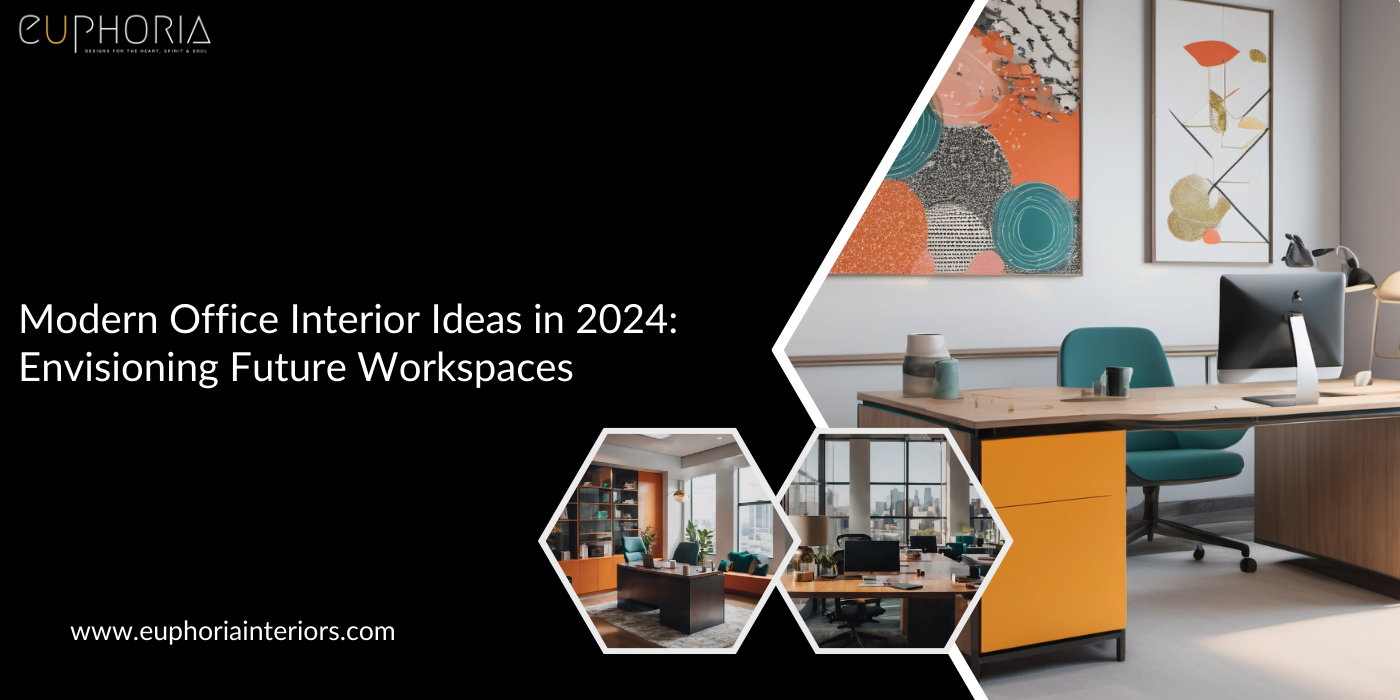This image, sourced from www.euphoriainteriors.com, showcases Modern Office Interior Ideas in 2024, Envisioning Future Workspaces. On the left side of the rectangular image, there's a black background with white text reading "Euphoria" at the top, followed by "Modern Office Interior Ideas in 2024: Envisioning Future Workspaces" and the website link at the bottom. The right side is divided by a white angled line and features a large photo and two smaller hexagon-shaped photos with white borders, presenting different interior design styles.

In detail, the largest photo features a light-colored wood desk with a waterfall edge and a yellow drawer cabinet. Positioned at the desk is a blue chair, and the backdrop consists of white walls adorned with two paintings, creating a clean and motivating workspace atmosphere. The floor is beige, enhancing the bright and welcoming feel. The top-left hexagon photo displays a dark desk facing an open window, accompanied by an orange bookshelf against the back wall. The middle hexagon showcases a brown wooden desk set before a large window with a cityscape visible in the background. Collectively, these designs provide diverse, efficient, and aesthetically pleasing office setups aimed at improving workplace feng shui and productivity.